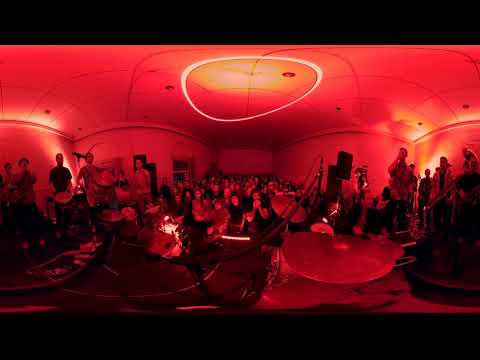The image captures an intense and intimate punk rock concert unfolding in a small, tight room, illuminated predominantly by vibrant red lights with hints of orange and yellow around the ceiling light sources. To the left, band members can be seen energetically playing their instruments, including guitars and drums, while the lead singer belts out lyrics off to the right. In the center, a lively mosh pit showcases the crowd’s enthusiasm, with a large number of tightly packed audience members contributing to the rowdy and high-energy environment. The scene is set indoors, possibly in a club, with a black border framing the photo, and no noticeable text present. The overall ambiance of the space feels closed-in and intensified by the converging walls and red hue dominating the view, enhancing the feeling of a powerful live performance.